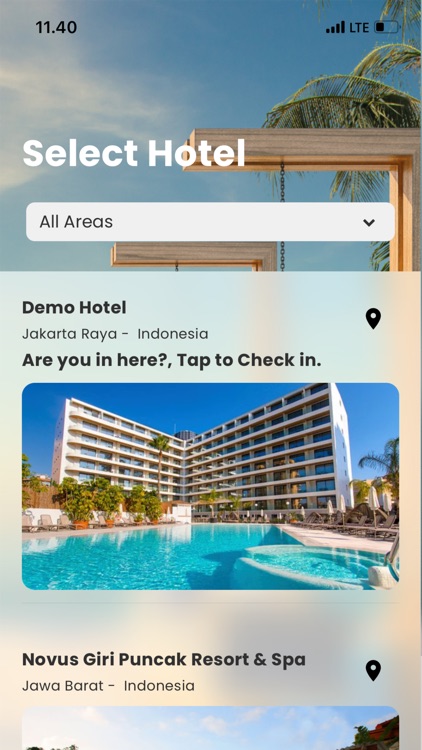This rectangular portrait image, resembling the shape of a smartphone screen, appears to be a screenshot from a mobile device. The image is divided into distinct sections, each containing detailed elements.

**Top Section (40% of the image):**
- In the upper left corner, the time "11:40" is displayed in black text.
- In the upper right corner:
  - A battery icon, approximately 35% filled, is positioned on the far right.
  - Next to it, the letters "LTE" are in uppercase.
  - To the left of "LTE," four black ascending bars indicate signal strength.
- The background features a sky with some visible palm tree tops and wooden structures.
- Left-aligned text displays "Select Hotel" in a large, white font.
- Below this text, there is a long white search bar:
  - On the left of the search bar, "All Areas" is written in dark gray.
  - On the right side, a downward-facing arrowhead indicates a drop-down menu.

**Middle Section (Another 40% of the image):**
- The first hotel, immediately beneath the search bar, is detailed with:
  - The name "Demo Hotel" in bold, left-aligned in the upper left corner.
  - Below the hotel name, "Jakarta Raya - Indonesia" is left-aligned.
  - Further down, in bold font: "Are You In Here?" followed by "Tap to check in."
  - An icon resembling a map pin drop is near the upper right corner of this section.
- Beneath the text, there's a landscaped rectangular image with rounded corners:
  - It shows a light blue pool in the foreground.
  - A six- or seven-story resort hotel is visible in the background, angled with the center deeper and the sides angled toward the viewer.
  - On the left side, there are some trees, and on the right, beach chairs are visible.
  - The entire scene is devoid of people.

**Bottom Section (20% of the image):**
- The second hotel, occupying the bottom part of the image:
  - The hotel's name: "Novis Giri Puncak Resort & Spa" (the ampersand symbol is used).
  - Below the hotel name: "Jawa Barat - Indonesia."
  - A black map pin drop icon is shown to the right of the text.
  - The very top sliver of the accompanying image is visible, showing a blue sky with white clouds, some tree tops on the left, and a hint of a building on the right.

Overall, the image provides a comprehensive layout of a mobile screen interface, highlighting two distinct hotels with their details and visuals.